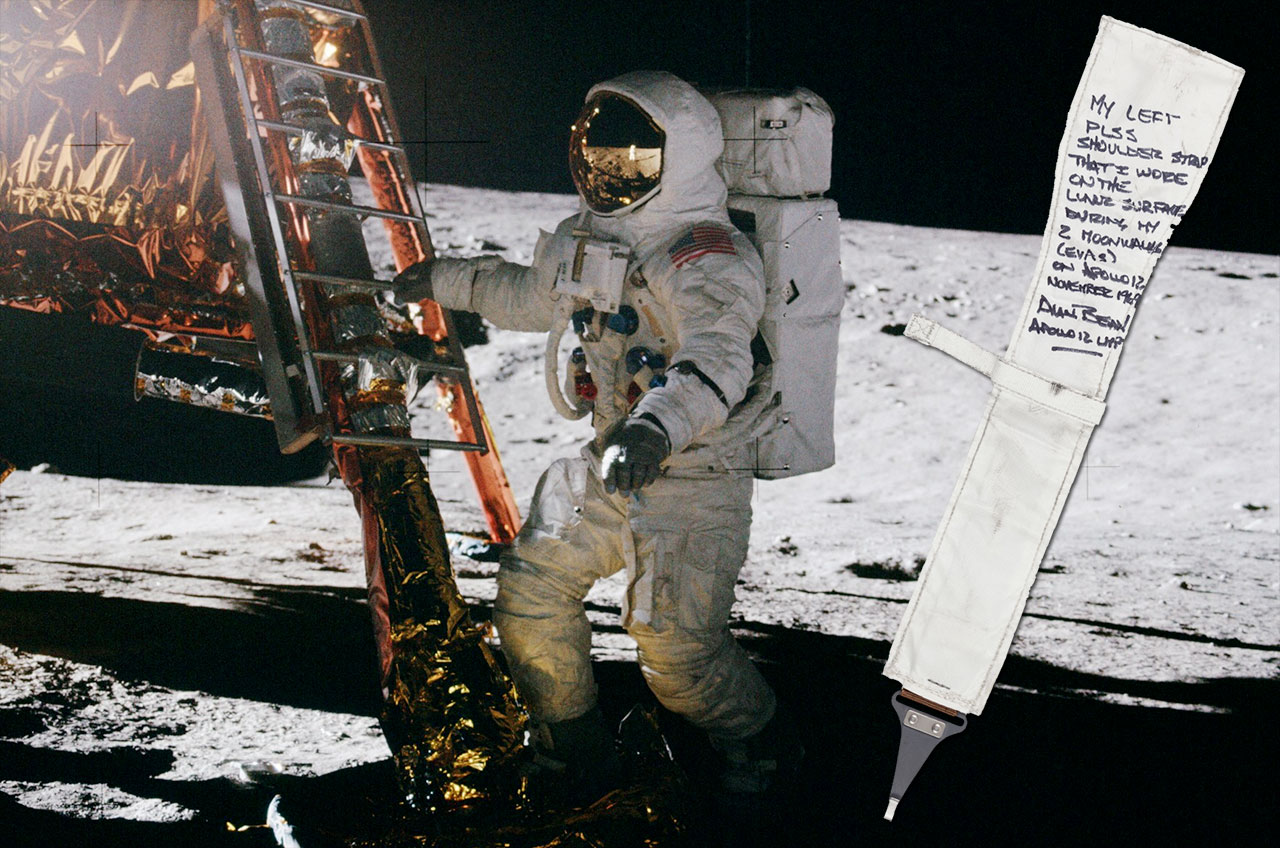This color photograph captures a historic moment as an astronaut, dressed in a white spacesuit adorned with a reflective visor and a red American flag on the left shoulder, climbs down from the lunar module onto the shadowy lunar surface. Positioned in the center of the frame, the astronaut has his right hand gripping a rung of the ladder affixed to the module's leg while one foot rests on the lower landing pad. His left hand extends outward. The lunar module, characterized by its gold and black insulation, fills the left side of the image, with the lunar surface and shadows surrounding the astronaut. On the right side of the photo, an overlaid white strap bears the inscription: "my left PLSS shoulder strap that I wore on the lunar surface during my two moonwalk EVAs on Apollo 12, November 1969." Below this, partially obscured text reads, "Apollo 12 something," indicating that this strap was worn on the moon by the astronaut during the Apollo 12 mission. The strap’s addition to the photo emphasizes its significance as a piece of lunar history.